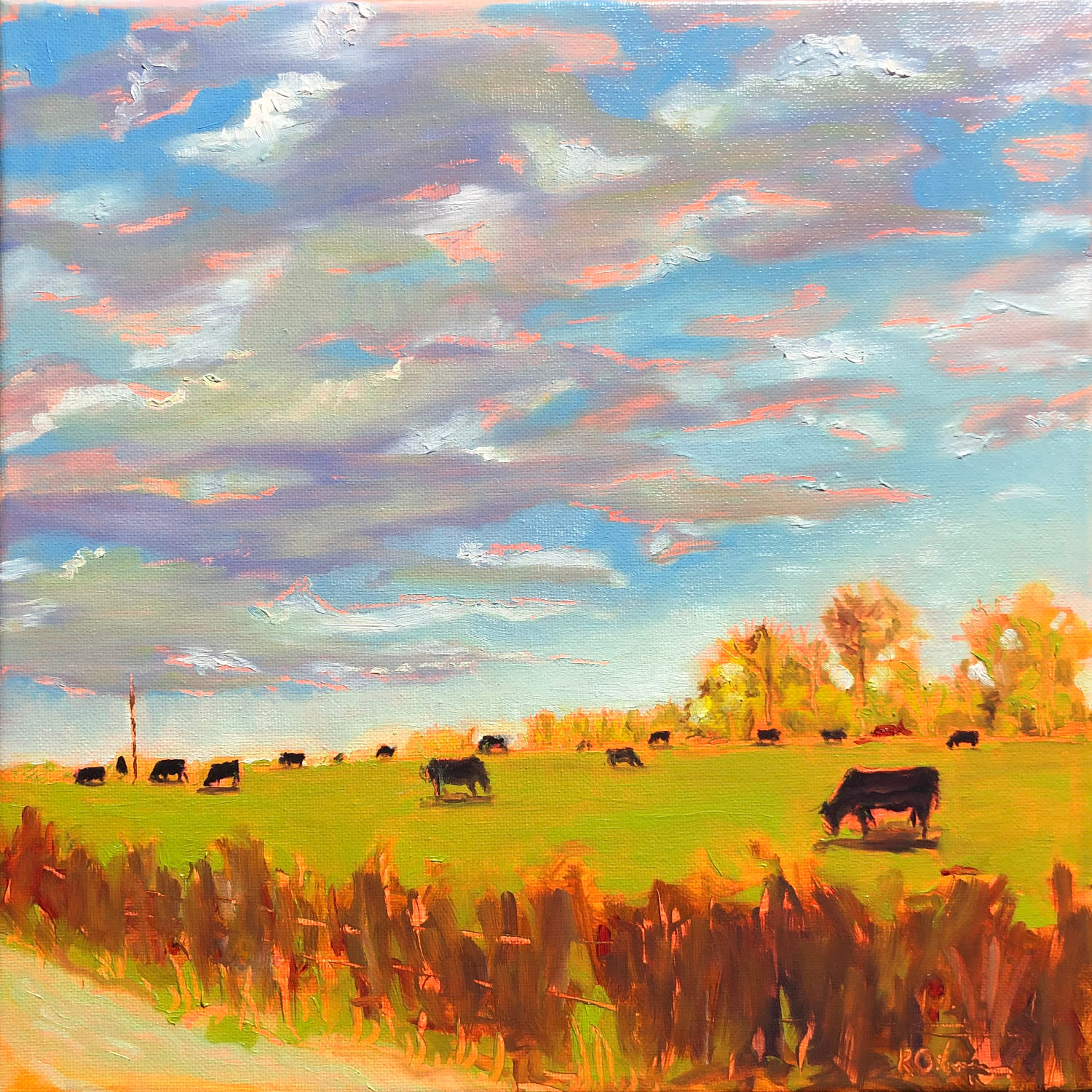The image is a square, abstract oil painting of a vibrant farm scene under a striking, colorful sky. The sky is a blend of deep blue, white, pink, purple, and dark grey hues. The clouds are tinged with gold and purplish colors, adding to the dynamic atmosphere. The foreground features a grassy area interwoven with lime green and gold, dotted with various brown and black cows, all of whom are milling around and eating the grass. A thin, light green and yellow road snakes from the bottom left corner, running alongside a wooden fence with shades of browns, reds, and orangey strips of wood, extending from left to right. Behind the field, there's a tree line in greens, yellows, and browns. Light pastel colors dominate the painting, giving it a muted yet serene feel. In the bottom right corner, the artist's initials, R, O, V, or L, are visible, adding a personal touch to the pastoral scene.